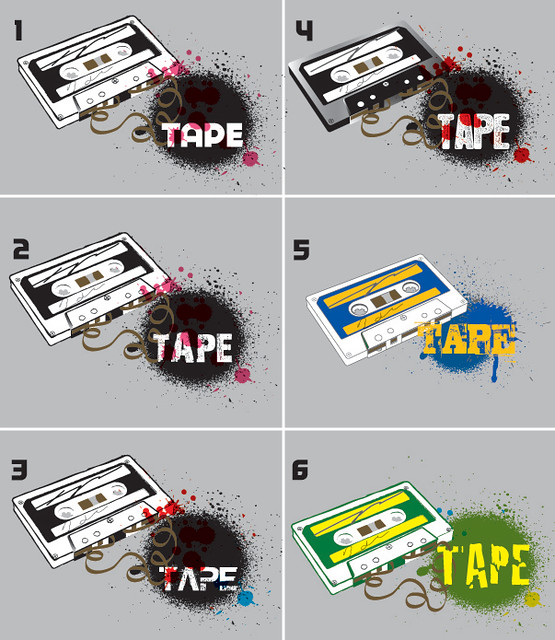The poster is an illustrated, vertical rectangle, featuring a series of six gray-background sections, each containing an image of a cassette tape. Numbered sequentially from one to six, each section showcases variations of the cassette and surrounding design elements. In the top left section (1), a black and white cassette tape is displayed with some of its tape unraveled and a black, paint-splash-like spot in the lower right corner, with the word "tape" inscribed in white. This scene is echoed in section two, with slight differences and additional red splotches. Sections three and four are nearly identical to section two, with very minimal changes. In section five, the cassette tape is depicted in blue and white, with the tape wound inside, and the paint splotch is now blue with the word "tape" in yellow. Finally, section six presents a green and white cassette with the tape pulled out, featuring a green paint splash with "tape" in yellow. Each image captures subtle variations of the cassette and design elements, creating a cohesive yet varied visual narrative across the poster.